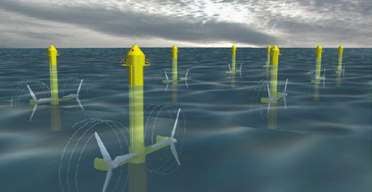The image is a 3D illustration depicting a water-based structure resembling reversed wind turbines. It consists of a series of at least eight tall, yellow poles positioned underwater, extending out in two rows across a bluish-gray body of water. Each pole features multiple white fanged blades, arranged in triplets on each end, mirroring the design of a wind turbine’s propellers. The water is transparent enough to reveal the continuation of these poles beneath the surface, where the propellers appear to be in motion, indicated by circular motion lines. The background showcases a cloudy sky with shades of white and gray, forming about the top third of the rectangular image. Despite the graphic's apparent low resolution and blurry quality, the details of the yellow poles, underwater blades, and their placement within the aquatic environment are clearly observable.